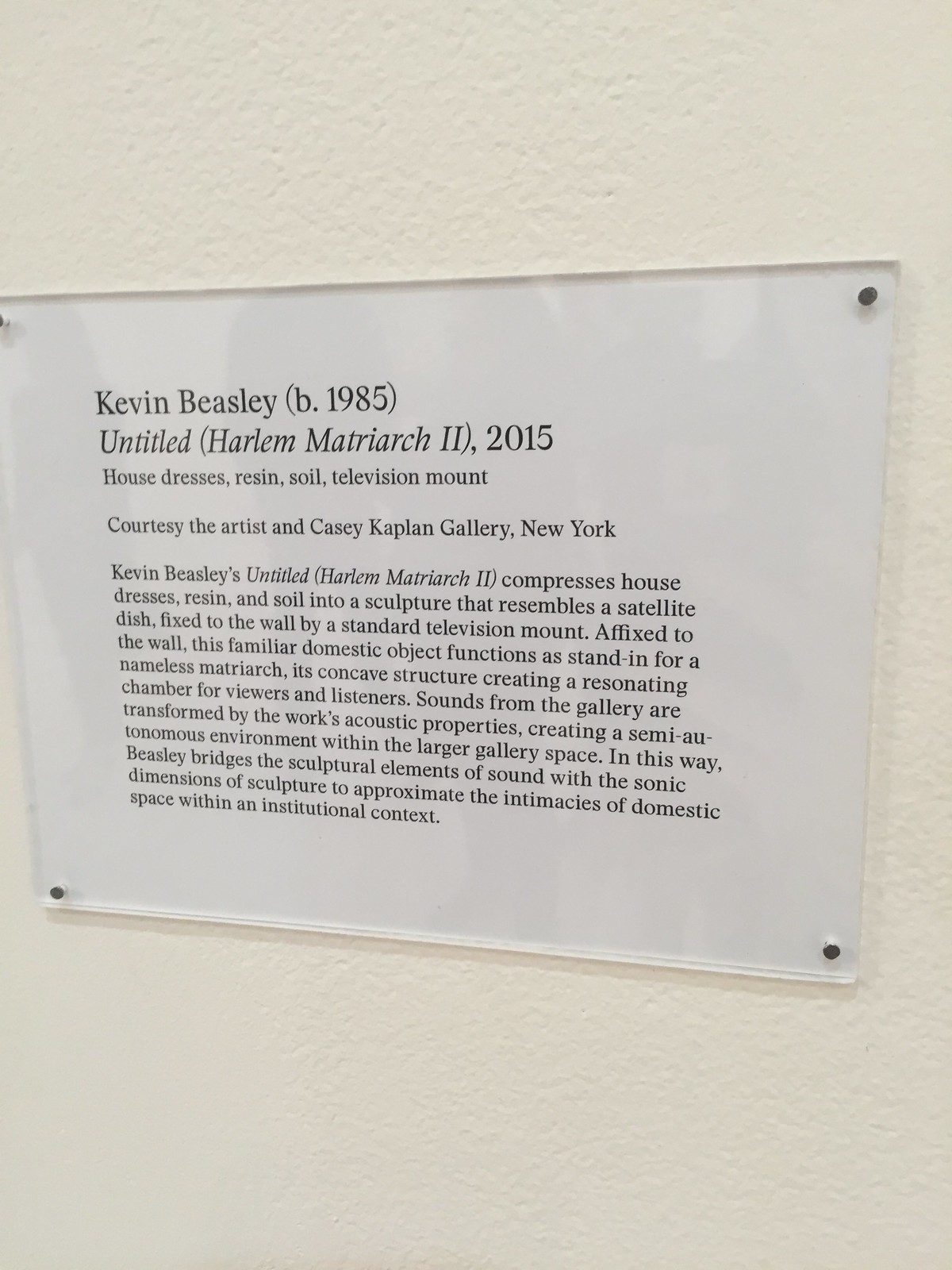This image showcases a white sign encased in plastic, affixed to a white wall, featuring black lettering. It serves as a label for an artwork by Kevin Beasley, born in 1985, titled "Untitled (Harlem Matriarch II)," created in 2015. The text describes the materials used in the piece: house dresses, resin, soil, and a television mount, and credits are given to the artist and the Casey Kaplan Gallery, New York.

Kevin Beasley's "Untitled (Harlem Matriarch II)" combines house dresses, resin, and soil to form a sculpture resembling a satellite dish, mounted on the wall using a standard television mount. This domestic object symbolizes a nameless matriarch, its concave structure acting as a resonating chamber that transforms sounds from the gallery into a unique acoustic experience. The work blurs the boundaries between sculpture and sound, echoing the intimacies of domestic life within the formal setting of a gallery.